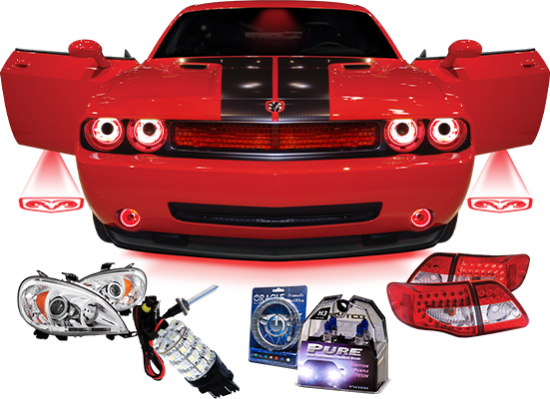The image features a digitally enhanced, bright red sports car with thick black racing stripes on its hood and various black accents. The car doors are open, revealing light projections that display the car's logo, resembling rams, onto the white background beneath. Surrounding the car, there are additional parts and add-ons showcased, such as headlights, a lighted steering wheel, and various other enhancements. Directly below the car, there are boxes labeled "Pure" in white and "Oracle" in blue. The entire scene appears to be set against a transparent background, possibly suggesting a promotional or stylized photo used for advertising purposes.